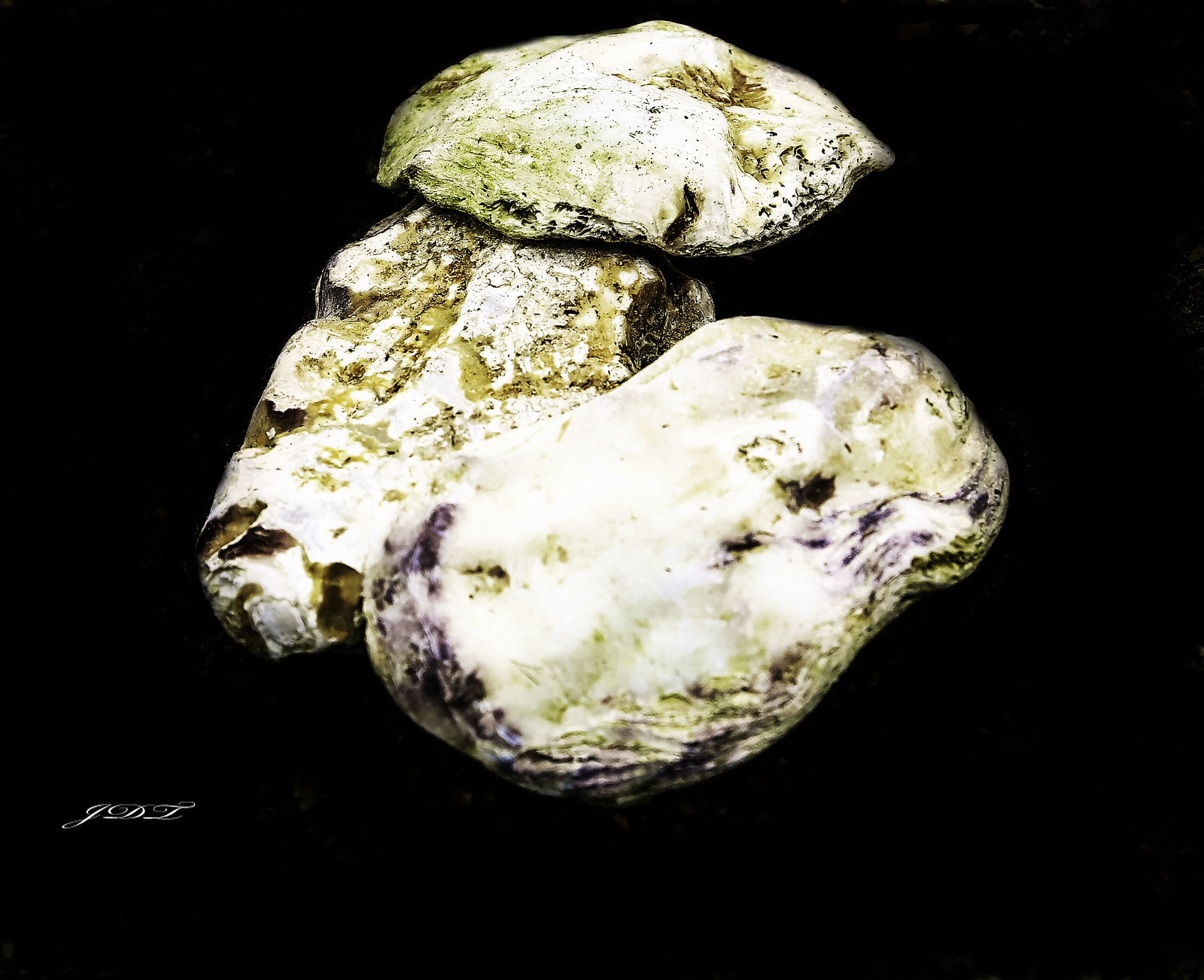In the foreground of this detailed close-up photograph, three rocks are positioned against a smooth, black background which enhances their features. The central rock has another horizontally-aligned rock balanced on top of it. In front of this central arrangement lies a third rock. All three rocks share a similar appearance, with rough textures marked by grooves and a sprinkling of moss. They display a mix of white, brown, and purple hues, with noticeable striations and pockmarks that add to their rugged character. The central rock, resembling an elongated potato, has smooth areas interspersed with rougher sections. In the lower left corner of the image, the initials "JDL" appear in white, cursive script, adding an artistic touch to the photograph.